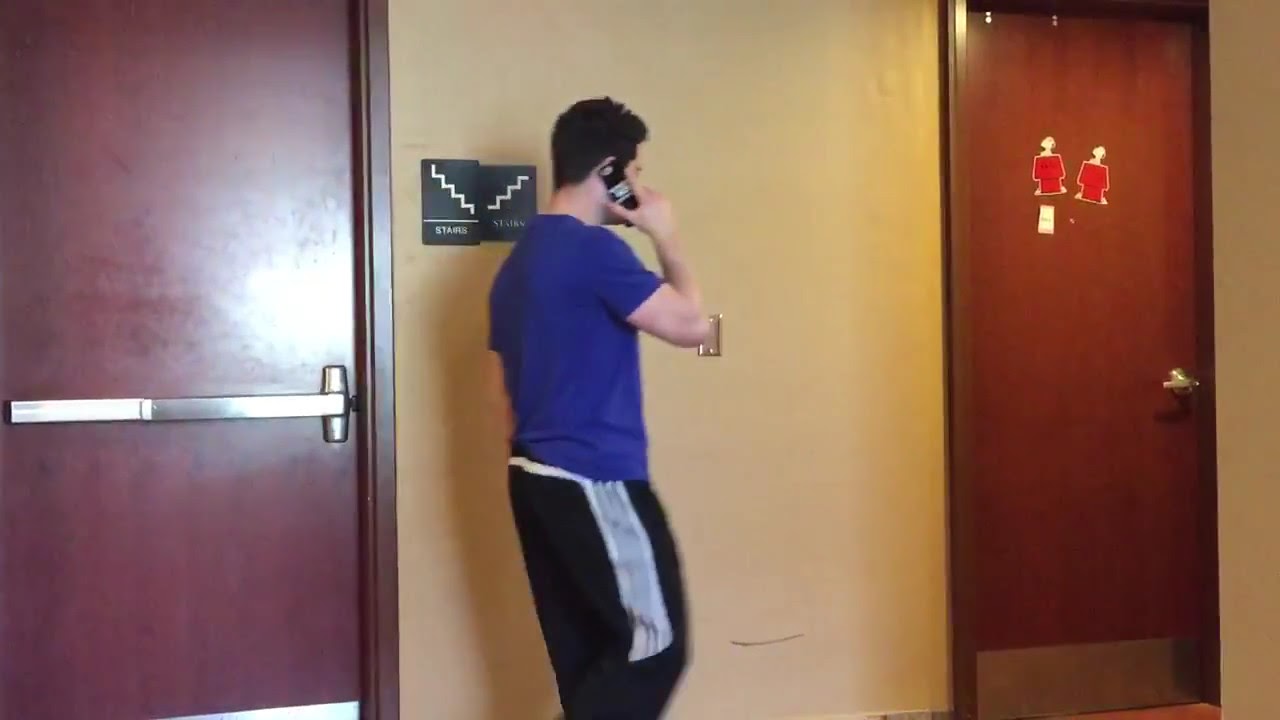This is a photograph of a Caucasian man with short dark hair walking away from the viewer towards the right side of the image, captured from a rear side angle. He is using his right hand to hold a black phone to his ear. He is dressed in a royal blue short-sleeved t-shirt and black pants that feature white stripes down the sides. The man is situated in a corridor with a yellowish-tan wall behind him. On the wall, near the left side of the photograph, are two black square signs featuring white zigzag lines indicating stairs, accompanied by the word "STAIRS" in white lettering beneath each zigzag. To the left of the man is a brown door with a silver push handle in the middle, while to his right is another brown door with a silver turn handle. The right door is adorned with two images of Snoopy on top of his red doghouses, visible from the shoulders up. The man is positioned between these two doors, enhancing the depiction of his surroundings.